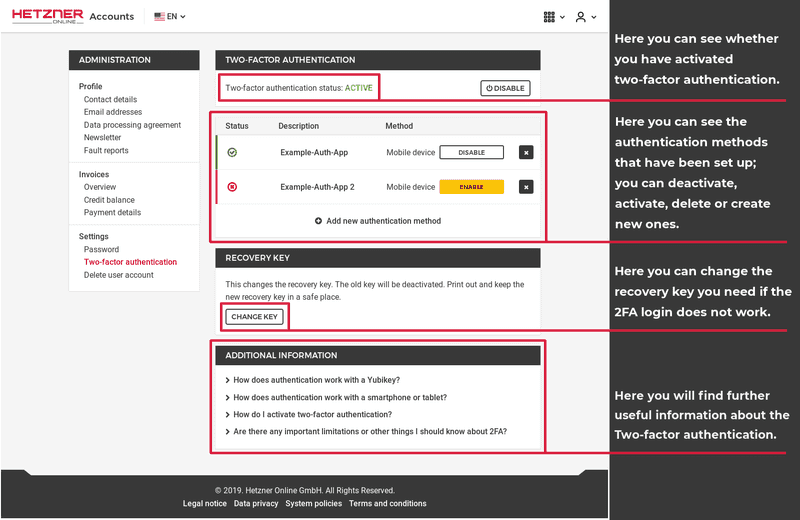**Caption:**

The screenshot captures Hetzner Online's website interface, identifiable by the "Hetzner Online" logo positioned in the top left corner, where "Hetzner" is rendered in red and "Online" in smaller black font. Adjacent to the logo, the "Accounts" section and a language selection option currently set to English are displayed against a white background.

On the far right of the top header, various navigational options presumably for different categories and account settings are visible. Scrolling down to the main content of the page, a greyish-white background features several sections organized into black and white boxes.

On the leftmost side, a black box titled "Administration" sits atop a white box containing relevant sub-menus. The sub-menu options under "Profile" include "Contact Details," "Email Addresses," "Data Processing Agreement," "Newsletter," and "Fault Reports." The "Invoices" section offers "Overview," "Credit Balance," and "Payment Details." Lastly, "Settings" encompasses "Password," "Two-Factor Authentication," and "Delete User Account," with "Two-Factor Authentication" currently selected.

Expanding the "Two-Factor Authentication" section reveals a detailed interface. A black box at the top reads "Two-Factor Authentication," followed by a white box with information in black font. Here, the two-factor authentication status is marked as active, with a button available to disable it. Below this, a table provides details with columns for "Status," "Description," and "Method," showcasing two examples. One method, "example-auth-app," is active (indicated by a black checkmark) and utilizes a mobile device. The other, "example-auth-app2," is disabled (highlighted by a red cross), also linked to a mobile device, with an option to enable it indicated by a yellow button and a black and white interface.

Further down, users can add a new authentication method. The section on recovery keys features a black box titled "Recovery Key" with a description in a white box below. It stresses the importance of securely storing the new recovery key after changing it, with a button labeled "Change Key." Lastly, additional information is provided in a white box titled "Additional Information," addressing how to authenticate using YubiKey, smartphones or tablets, activate two-factor authentication, and understand its limitations.

Each section is outlined in red, providing guidance on their purpose. For instance, the "Two-Factor Authentication Status" box clarifies if the feature is active. Another box explains the table for "Status, Description, and Method," detailing how to manage authentication methods. The "Change Key" button's function is outlined, along with a box for "Additional Information" detailing all relevant aspects of two-factor authentication.